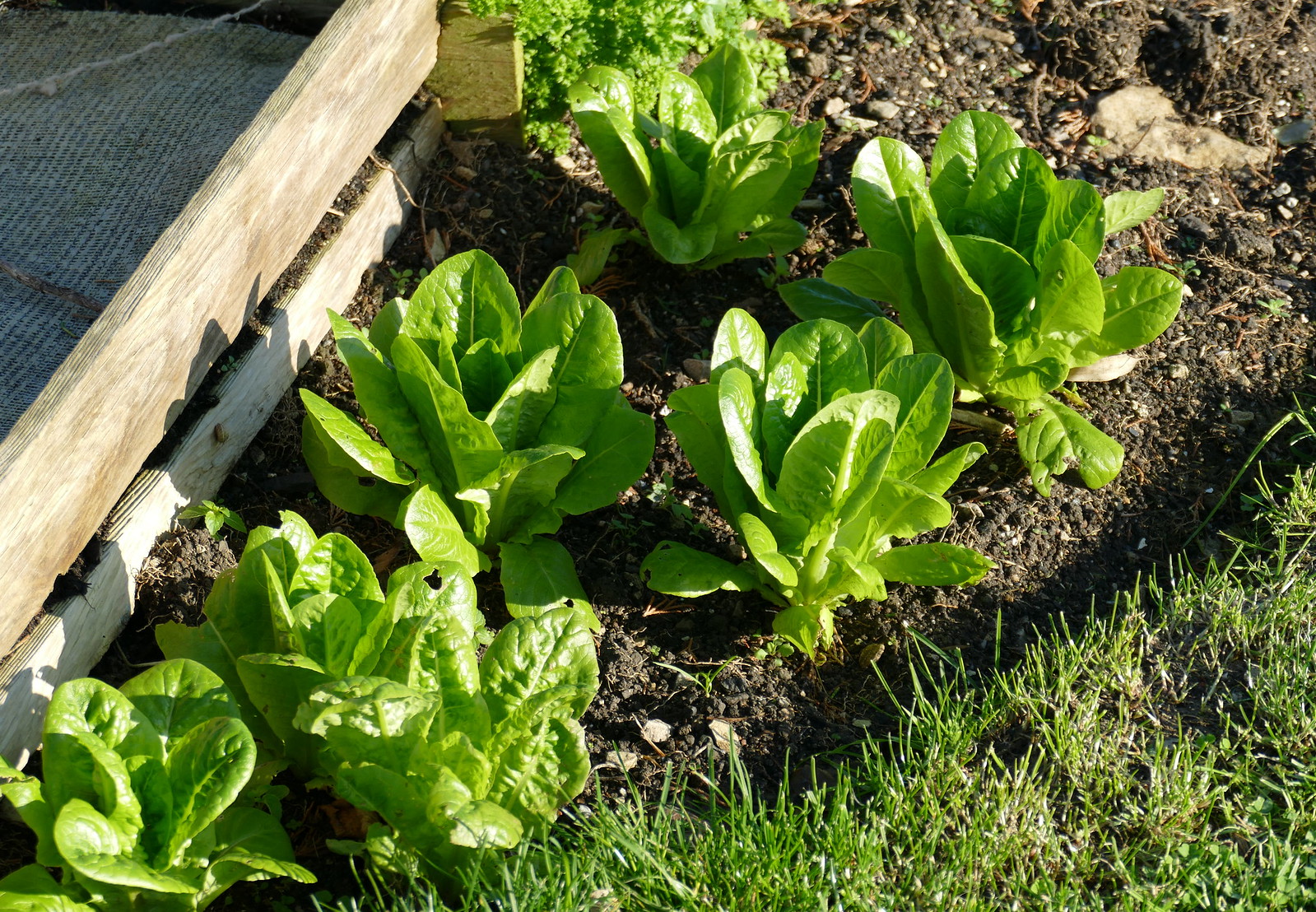This daytime color photo, taken from an elevated perspective, captures a small garden plot adjacent to a patch of grass. The focal point of the image is seven green spinach plants, arranged in a staggered pattern rather than in neat rows, thriving in rich soil. On the left side of the garden bed, there is a wooden structure resembling a filter box, presumably used for sifting rocks from the soil. The lush green foliage of the spinach, noticeably distinct and vibrant, suggests they are about three and a half weeks away from harvest. The bottom right corner of the image features a triangular section of green grass, framing the scene.